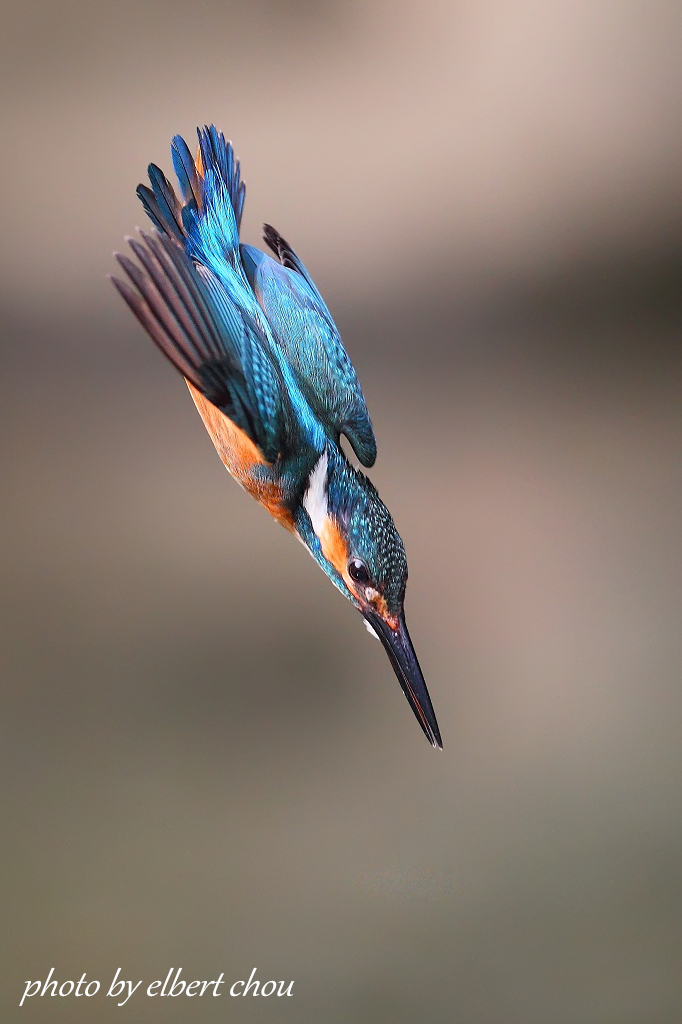The photograph by Albert Chou, noted in white italicized font at the bottom left corner, captures a small, iridescent blue bird in mid-dive, presumably aiming for food with a determined gaze. Its body, ranging from dark navy to a shimmering light blue, features an orange underbelly and orange cheeks. The bird has a noticeably long, sharp beak and is shown in a precise downward angle, indicating high speed and purpose. The background is entirely blurred, blending gray, black, and brown hues, effectively highlighting the bird's vivid colors and fast motion.